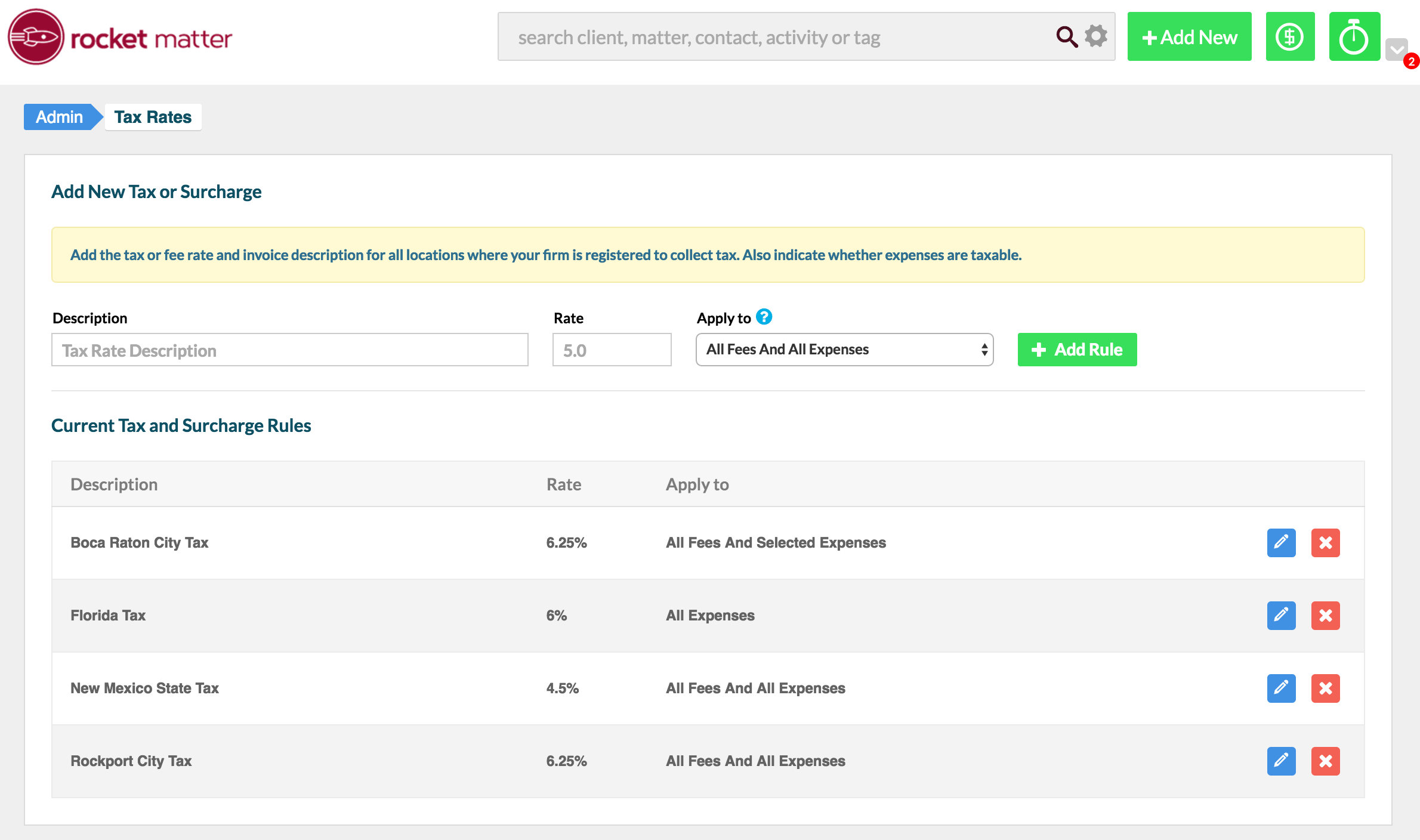The image depicts a user interface design with various elements and buttons on a white background. 

In the top left corner, there is a simplistic, childlike circular rocket ship logo in white. Adjacent to the logo, "Rocket Matter" is written in black text. To the right, there is a gray search bar displaying the placeholder text "Search Client Matter Contact Activity or TAG" in gray.

On the right side, a green button labeled "Add New" sits next to icons of a dollar sign encased in a circle and a stopwatch, both on a white background. Below this, on a gray background, a blue button contains the word "Admin" and is accompanied by another button with a white checkmark and the text "Tax Rates" in black.

Further down, a section on a white background entitled "Add New Tax or Surcharge" features black text. Below this, against a light yellow background, instructions in black text read: "Add the Tax Fee or Rate Invoice Description for all locations where your firm is registered to collect tax. Also indicate whether expenses are taxable." 

The subsequent section displays a black background with labels in black reading "Tax Rate," "Tax Rate Exemption," "Rate" (noting 5%), and "Apply To," which includes a selectable option for "All Fees and All Expenses." Additionally, a green button labeled "Add Rule" in white is present.

Moving further down, a list of current taxes and surcharges is provided, detailing descriptions such as "Boca Raton City Tax," "Florida Tax," "New Mexico State Tax," and "Rockport City Tax." Associated with these are application options stating "Apply To," with choices like "All Fees and Select Expenses," "All Expenses," and "All Fees and All Expenses." On the right side, there is also a blue square with a white pencil icon and several red squares containing white Xs.

This detailed interface is richly populated with functional buttons and informative text, providing users with a comprehensive view and the ability to manage various tax-related settings and entries.